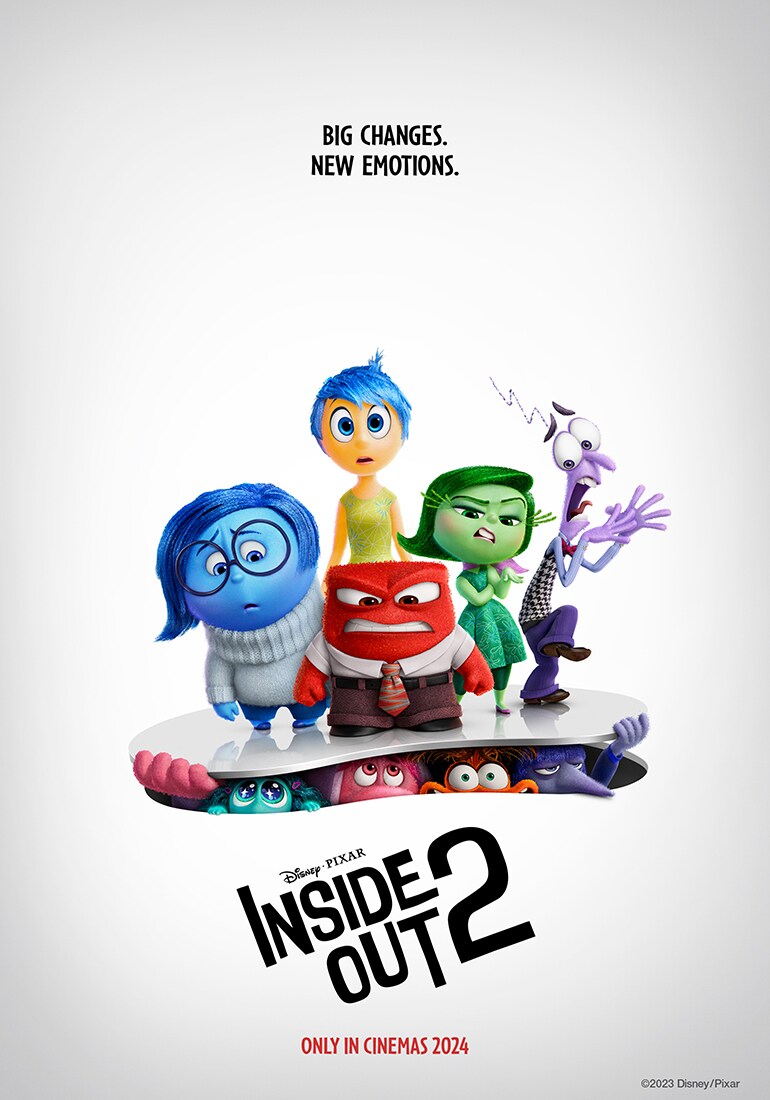This movie poster for Disney Pixar's "Inside Out 2," set to release exclusively in cinemas in 2024, features a predominantly white background. At the top of the poster, the text reads "Big Changes, New Emotions" in small black letters. The title "Inside Out 2" is prominently displayed at an angle from the lower left-hand corner upwards in black font, with "Disney Pixar" above it and "Only in Cinemas 2024" in red below.

In the center of the poster, five main characters from the original movie, representing different emotions, are vividly illustrated. These include a blue girl with blue hair and blue skin, a red character wearing a tie, button-down shirt, and brown slacks, a green girl with green hair and a green dress, a freaked-out looking purple character, and another blue-haired girl with fair skin and a green dress. They stand on a cutout stage, beneath which other characters—some visible with hands or noses peeking out—appear to be trying to escape, while the primary characters seem to be keeping them confined. At the bottom right of the poster, a small text notes "2023 Disney Pixar."